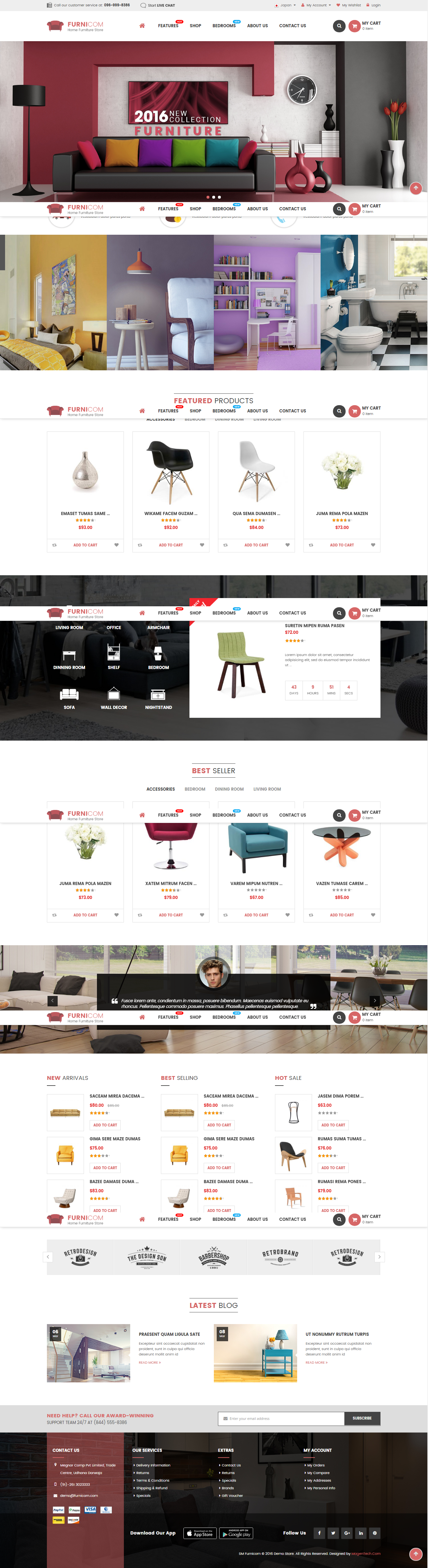This is a detailed caption for a smartphone screenshot of the Furniture.com website. The screenshot showcases multiple elements:

At the top of the screen, there are four banners prominently displayed. The first banner advertises the 2016 Furniture Collection, featuring a fully set up futuristic living room. This room includes a sofa adorned with six throw pillows, a lamp, a wall clock, and a photograph to illustrate the new collection. The living room also features a table with vases, adding to the modern aesthetic.

Below this banner, various sections are visible. To the left, there is an image of a complete bedroom setup. Adjacent to the bedroom is a cozy sitting area furnished with a chair and a small table. Right next to the sitting area is a shelving display, followed by a bathroom featuring black and white tile flooring, a toilet, and a double vanity.

Further down, the website showcases individual products that appear to include chairs, a light bulb, and other miscellaneous items. Another banner, displayed in black, features a single chair. Following this, there are more chairs and coffee tables. A subsequent banner shows a person's photograph along with a hardwood floor and a table surrounded by chairs, possibly depicting another living room or a different section of the sofa setup.

Near the bottom of the screenshot, additional individual items are displayed, accompanied by a section labeled "The Latest Blog," indicating the website's latest blog posts.

This comprehensive view provides an insight into the diverse furniture offerings and layout sections available on Furniture.com.